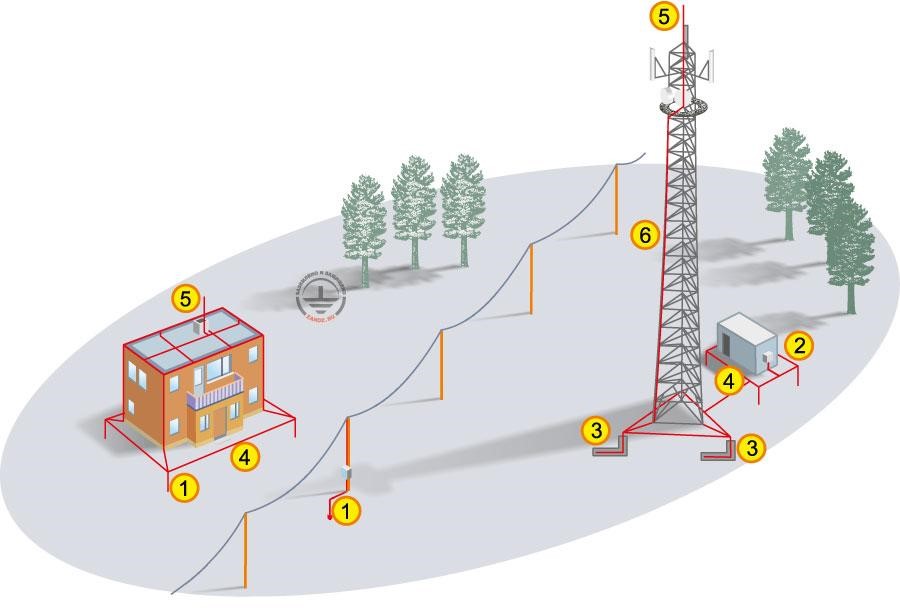The image appears to be a detailed diagram of a park or facility featuring prominent electrical and structural elements. Central to the diagram is a large steel lattice electrical tower labeled with the numbers three, four, five, and six, marked in little yellow circles with an orange rim. To the right of this tower is a small white building or generator, labeled with the numbers two and four. Adjacent to these, there is an orange building with a glass or potentially solar-paneled roof, situated at the top left edge of the image, and marked with the numbers one, four, and five. A chain-link fence runs vertically down the middle of the image, organizing the electrical lines and structures. Surrounding these elements, the diagram is dotted with six green pine trees, three on each side of the fence.